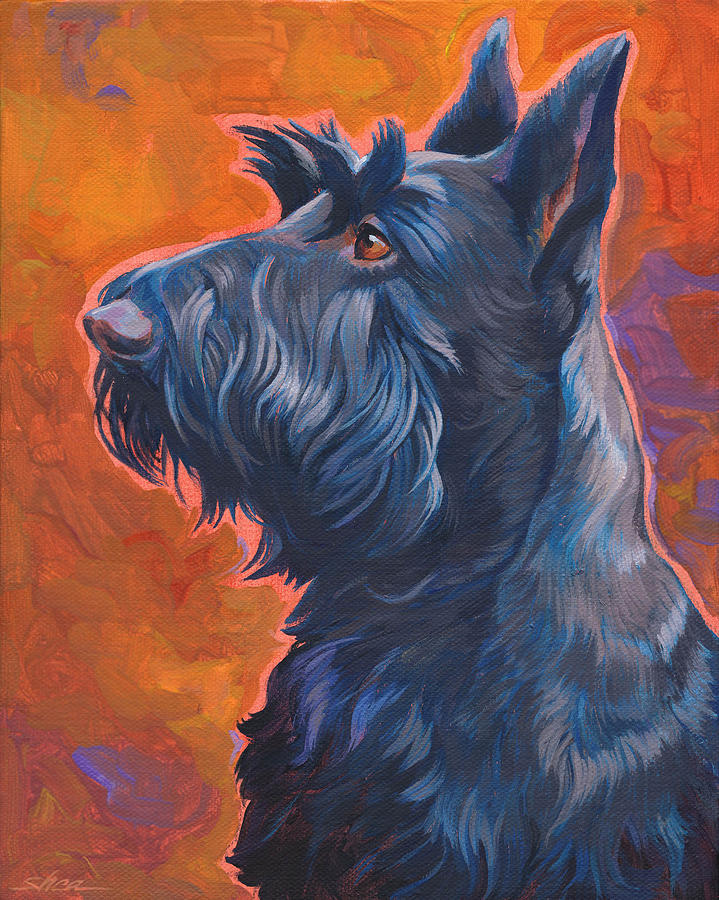This detailed illustration captures a profile view of a black terrier, possibly a West Highland Terrier, notable for its striking tufty eyebrows and upright, pointed ears indicating alertness. The terrier’s shiny black fur is subtly accented with blue highlights, and its amber-hued eyes are fixed on something off to the side, giving it a focused expression. The dog's profile reveals a jutted black nose and thick fur hanging between its eyes and nose, with the image showing the dog from the chest up, occupying the bottom right to the middle left of the painting. The swirling background is a vibrant blend of oranges and greens with hints of blues, pinks, and gray, creating a dynamic contrast that frames the terrier beautifully.